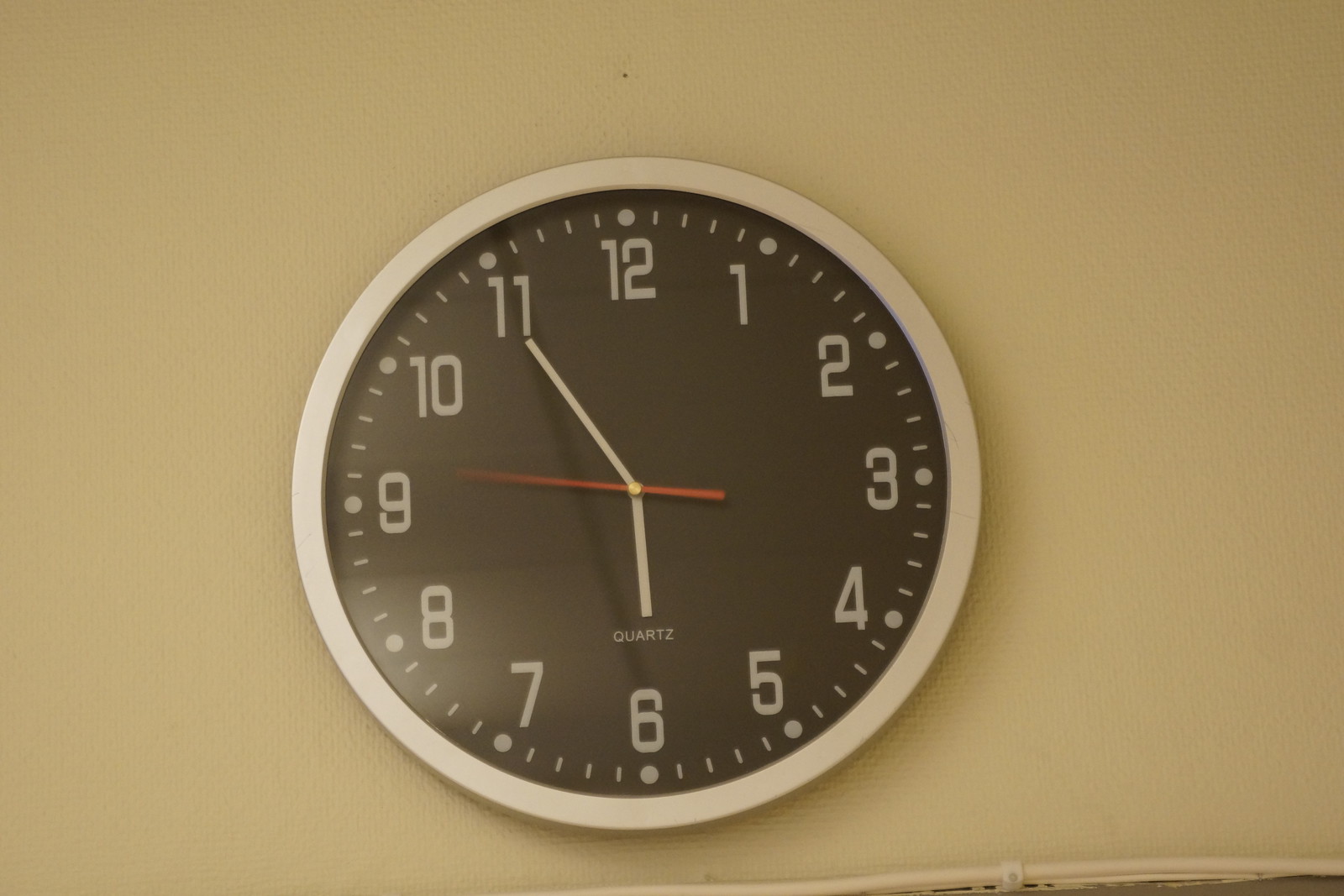The image depicts a simple, round, analog wall clock with a silvery white frame and a black clock face. The clock displays standard white numerals from 1 through 12 and white markings dividing the hours into 15-minute segments. The hour and minute hands are white, while the thin second hand is red. The time shown is approximately 5:54 or 5:55. Noteworthy features include the word "Quartz" printed above the 6 o'clock position and a slight shine visible on the bottom left side of the clock's frame. The clock is mounted on a wall that appears to be a dirty yellow or tan color. The overall setting is somewhat unremarkable, with the clock centered in a horizontal rectangular image, and wall space surrounding it.